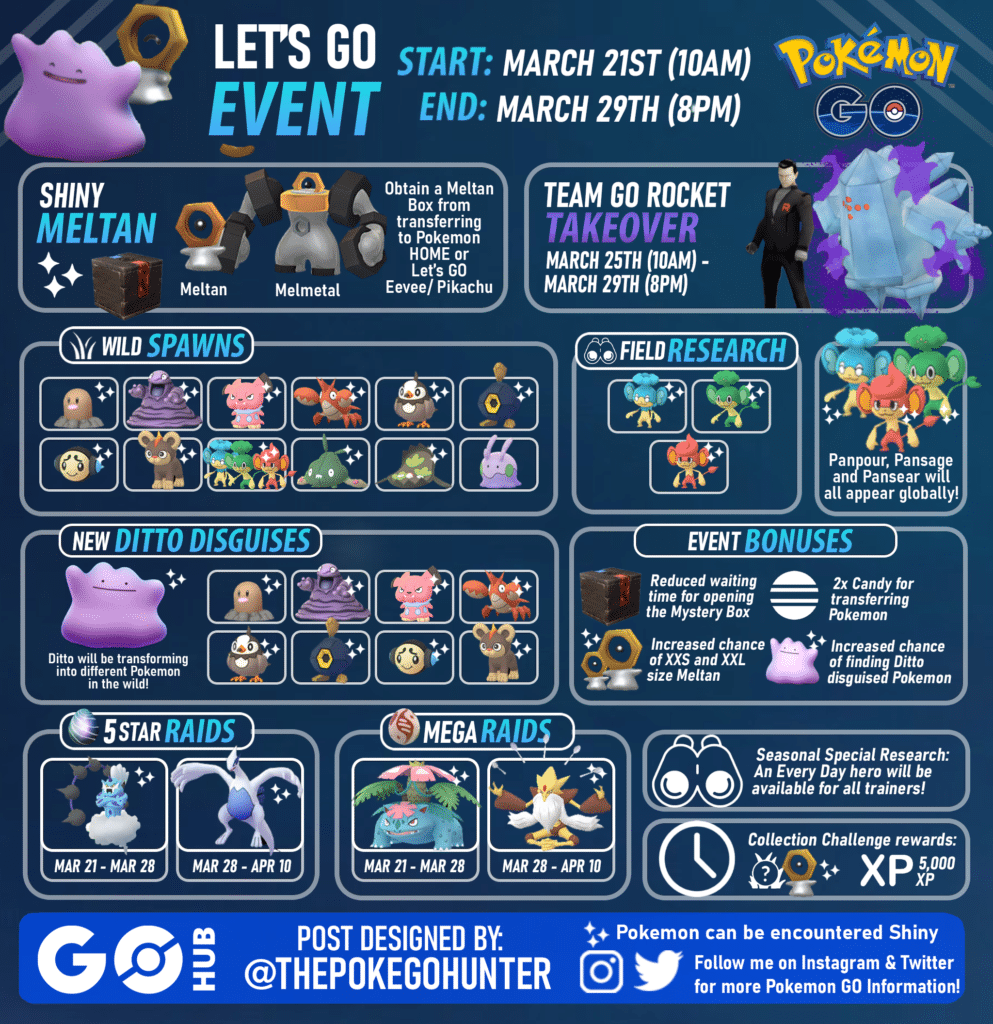This image appears to be an official promotional graphic for a Pokémon Go event that ran from March 21st to March 29th (year unspecified). The event features a plethora of activities and rewards, including the chance to encounter shiny Pokémon, engage in battles with Team Rocket bosses, and complete special field research tasks. Notable focal points of the event include unique spawns, various bonuses, and encounters with Ditto disguised as different Pokémon. It also highlights five-star raids and mega raids, offering players numerous opportunities for involvement.

The design has a dark blue to grey metallic background, adding a sleek and immersive feel. Various Pokémon are depicted, including recognizable ones like Ditto and Dugtrio, among others. The layout is meticulously organized, detailing how to obtain special Pokémon, the event’s bonuses, and specific start and end times. At the bottom, the image credits its creation to "PokeGoHunter" and mentions "GoHub," along with providing information on how to follow the designer on Instagram and Twitter for more updates on Pokémon Go and similar events.